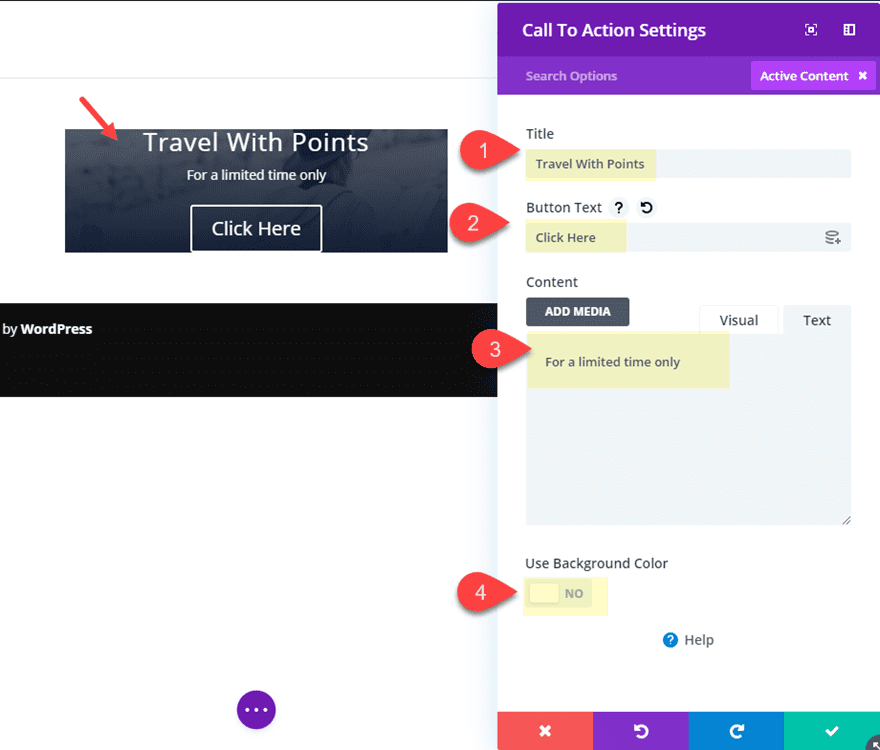In the image, we observe a square-shaped layout, although the exact dimensions are indistinct due to the white background that lacks clear edges. The image depicts a web application interface, with the right-hand side resembling the format of a mobile phone screen, occupying roughly 40% of the space.

At the top of this mobile screen mimic, there's a prominent purple banner featuring the text "Call to Action Settings" in white. Adjacent to this text, on the right, are two buttons: one that appears to be for expanding options and another that resembles a page icon.

Beneath the banner, there's a search options bar. This bar prominently displays the phrase "Search Options" in gray text. To its right, there's another section shaded in a lighter purple, encompassing the text "Active Content" followed by an 'X' icon, likely indicating a filter setting.

Further down, the background remains white. Here, a bold header labeled "Title" is followed by additional text, "Travel with Points." Nested within this section appears to be a search bar, which contains black text overlaying a tan background.

Additionally, the interface includes buttons and text content beneath the search bar, with options to "Use Background Color." There are also four distinguishable tabs positioned on the left side of these sections, labeled one through four, indicating different segments within the application.